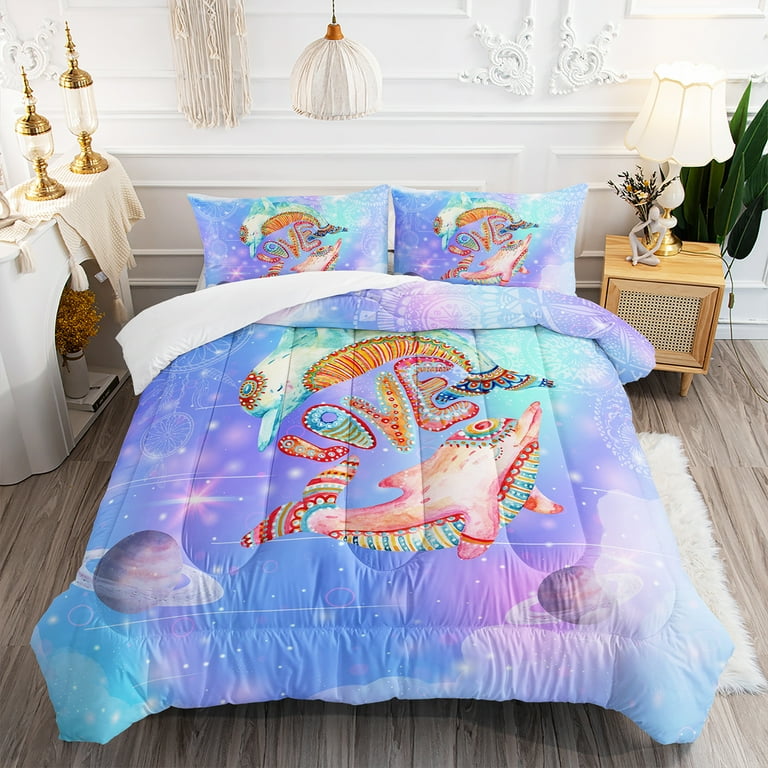The image depicts an ornate bedroom centered around a vividly colorful bed. The bedspread and matching pillows showcase a striking design of two dolphins, one light blue and the other pink, circling around the word "love" in red lettering. The dolphins, adorned with ornate bead patterns, swim amidst a cosmic scene with planets, stars, and a dream catcher, all set against a vibrant purple and blue background. On the right side of the bed, there’s a modern wooden nightstand with a white lamp. To the left, an ornate table holds two gold lanterns with white bulbs. The floor is brown hardwood, and the walls are white with decorative panels. The room also features a white-covered piece of furniture, possibly a fireplace, adorned with gold candles and a vase with flowers underneath. This blend of a cosmic bedspread in a sophisticated room creates a uniquely eclectic aesthetic.